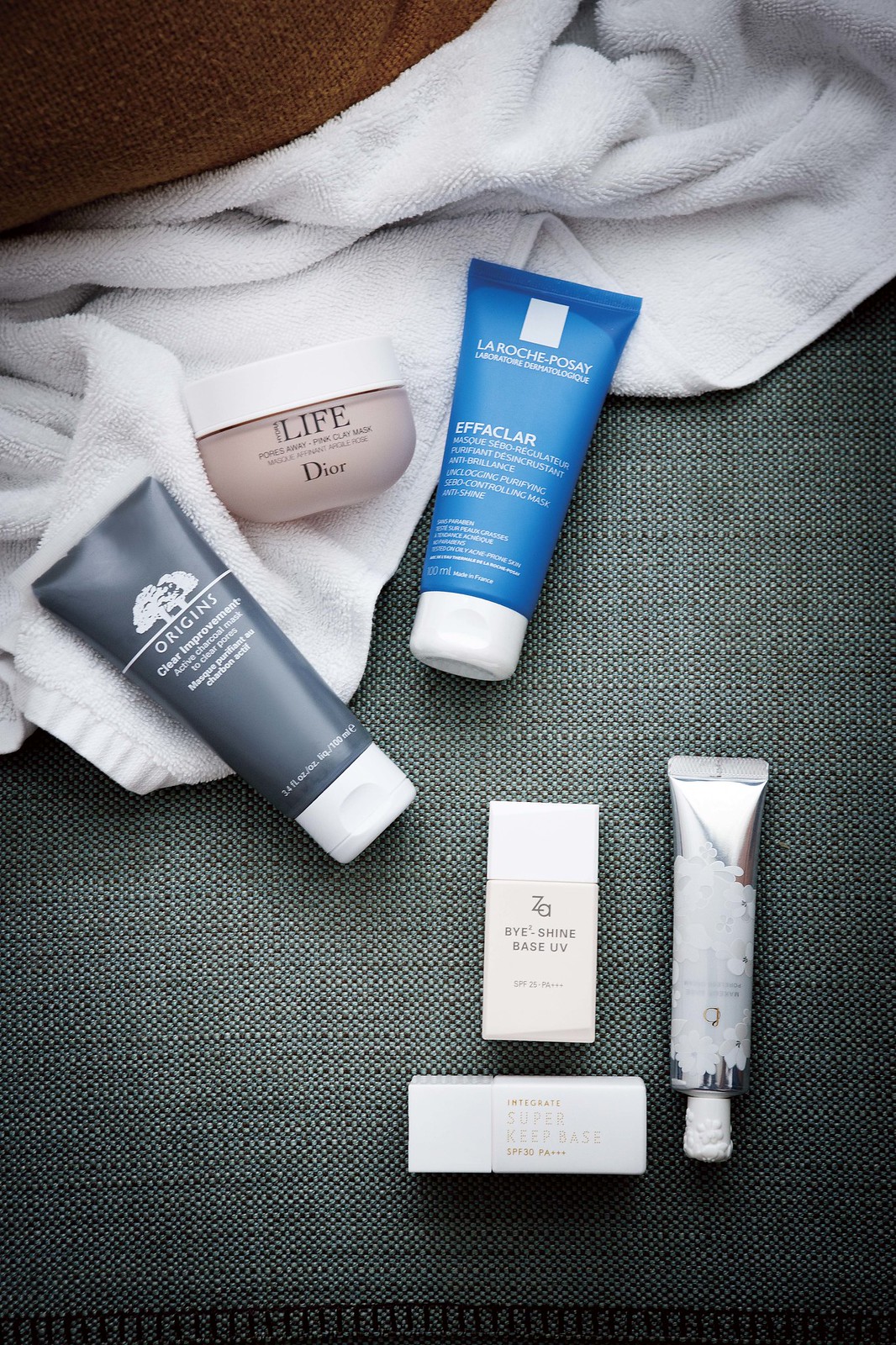This professional product photo showcases a comprehensive skincare routine set, meticulously arranged to highlight each product. Central to the set is a variety of skincare products, including items from well-known brands. 

Prominently displayed is a tube from Origins with the label "Clear Improvement," suggesting a product designed for deep cleansing and pore refinement. Adjacent to it, another product brandishes the name "La Roche-Posay," a renowned skincare brand, with the additional text "Anthelios XL UV" indicating sun protection features. Below these, a sunscreen tube further emphasized for its UV defense properties is also included in the set.

The right side of the image features a sleek, silver tube, adding a touch of modern elegance to the collection. The entire layout exudes a sense of both functionality and luxury, ideal for anyone looking to establish or elevate their skincare routine.